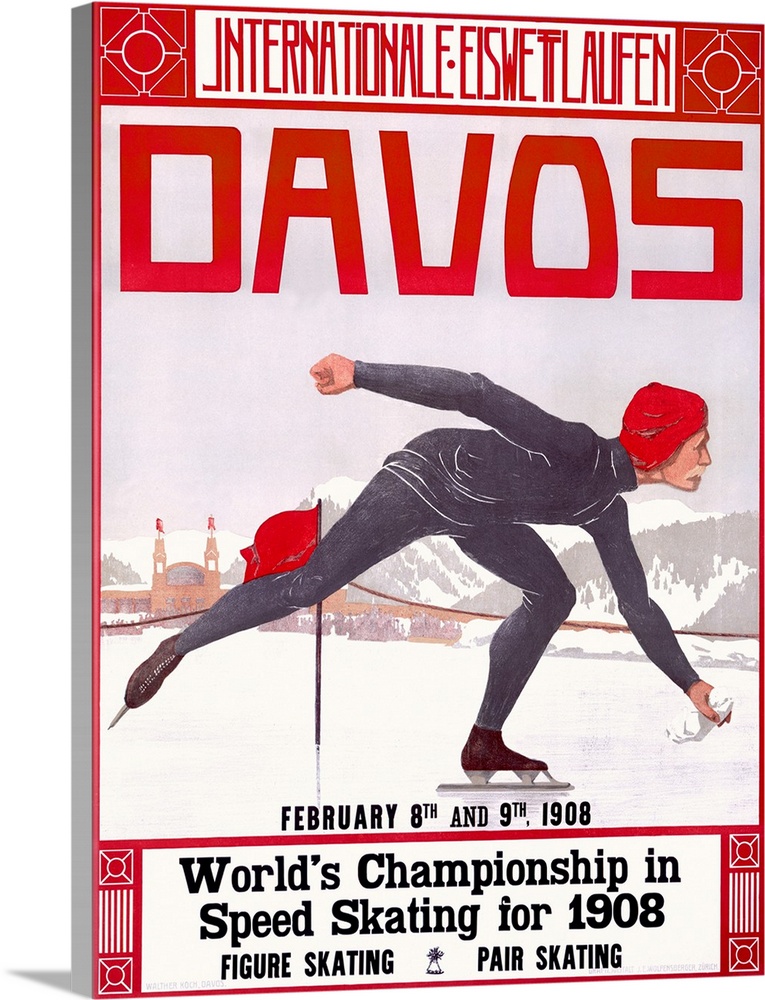The image depicted is a stylized poster from 1908 advertising the World Championship in Speed Skating, Figure Skating, and Pair Skating, held on February 8th and 9th in Davos. The poster features vivid red and white color tones, accented with grays and dark blues, and is fully bordered by a thin red outline. The central image displays an elderly man skillfully ice-skating outdoors, against a snow-covered backdrop with mountains and trees. He is dressed in a blue bodysuit, red hat, and gray turtleneck with matching pants, one leg raised and one arm extended back as if performing a trick or gaining speed. Above this figure, in large red letters, the words "Internationale Eislaufen" are prominently displayed, with "Davos" in massive capital letters below. The lower part of the poster contains black lettering that reads "World's Championship in Speed Skating for 1908," with additional mentions of "Figure Skating" and "Pair Skating."